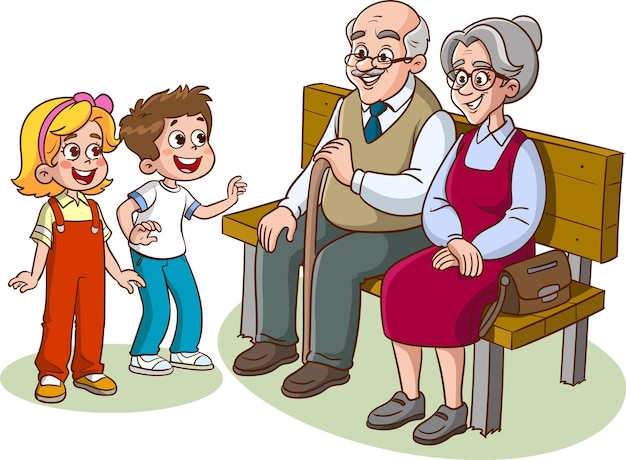The animated image features four cartoon-like characters on a solid white background. On the left, two small children are standing and smiling brightly. The girl, positioned on the far left, has shoulder-length blonde hair adorned with a pink bow. She wears a light green short-sleeved shirt under red overalls, complemented by orange shoes. Her cheeks are whimsically dotted with red. Next to her is a boy of the same height. He has brown hair and dark eyes, and is dressed in blue pants and a white shirt with blue cuffs and dark shoes.

On the right, two grandparent-like figures are sitting on a brown wooden park bench. The grandmother, on the far right, has gray hair styled up and wears glasses. She sports a dark red dress with a long-sleeved light purple shirt underneath and gray shoes. A brown purse is placed on the bench next to her. The grandfather, who is seated to her left, is bald on top with white hair on the sides. He wears glasses, a tan sweater vest over a light-colored long-sleeved shirt, a teal blue tie, greenish-blue pants, and brown shoes. Both grandparents are smiling warmly at the children. The floor under the characters consists of light green circles, adding to the cohesive and cheerful atmosphere of the scene.